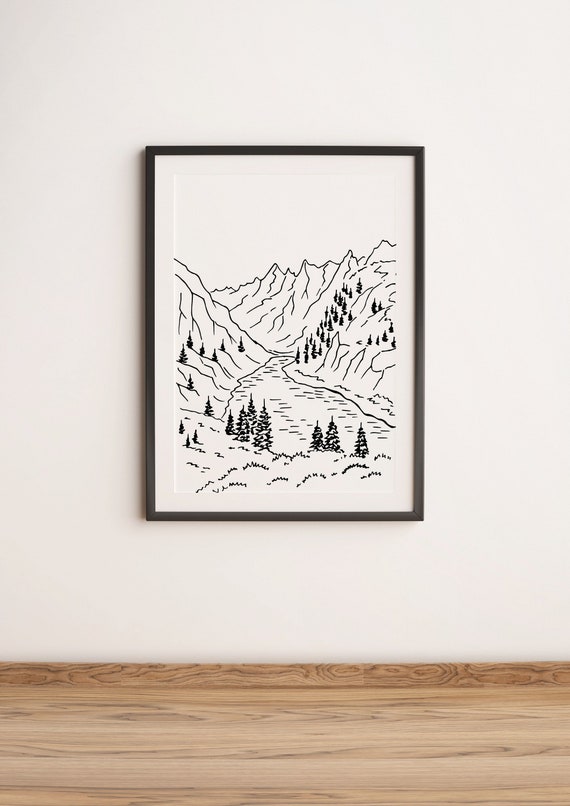This image captures a tightly framed black and white pen or ink drawing, elegantly encased within a slim black frame that includes a white mat. The artwork, hanging on a white wall above a light brown wooden floor, portrays a serene landscape scene. Central to the drawing is a wide-mouth river flowing between two prominent mountain ranges, progressing towards a more distant set of peaks on the horizon. The riverbanks in the foreground are adorned with evergreen trees, while sparse pines dot the left mountain, and a denser array of evergreens climbs the slope of the right mountain. The farthest mountain range remains bare, and the sky above is stark white, adding to the minimalistic yet detailed aesthetic. Wavy lines near the bottom of the artwork suggest patches of grass, enhancing the scene's natural charm. The planked oak flooring beneath the photo contributes to the overall warm, rustic feel of the display.